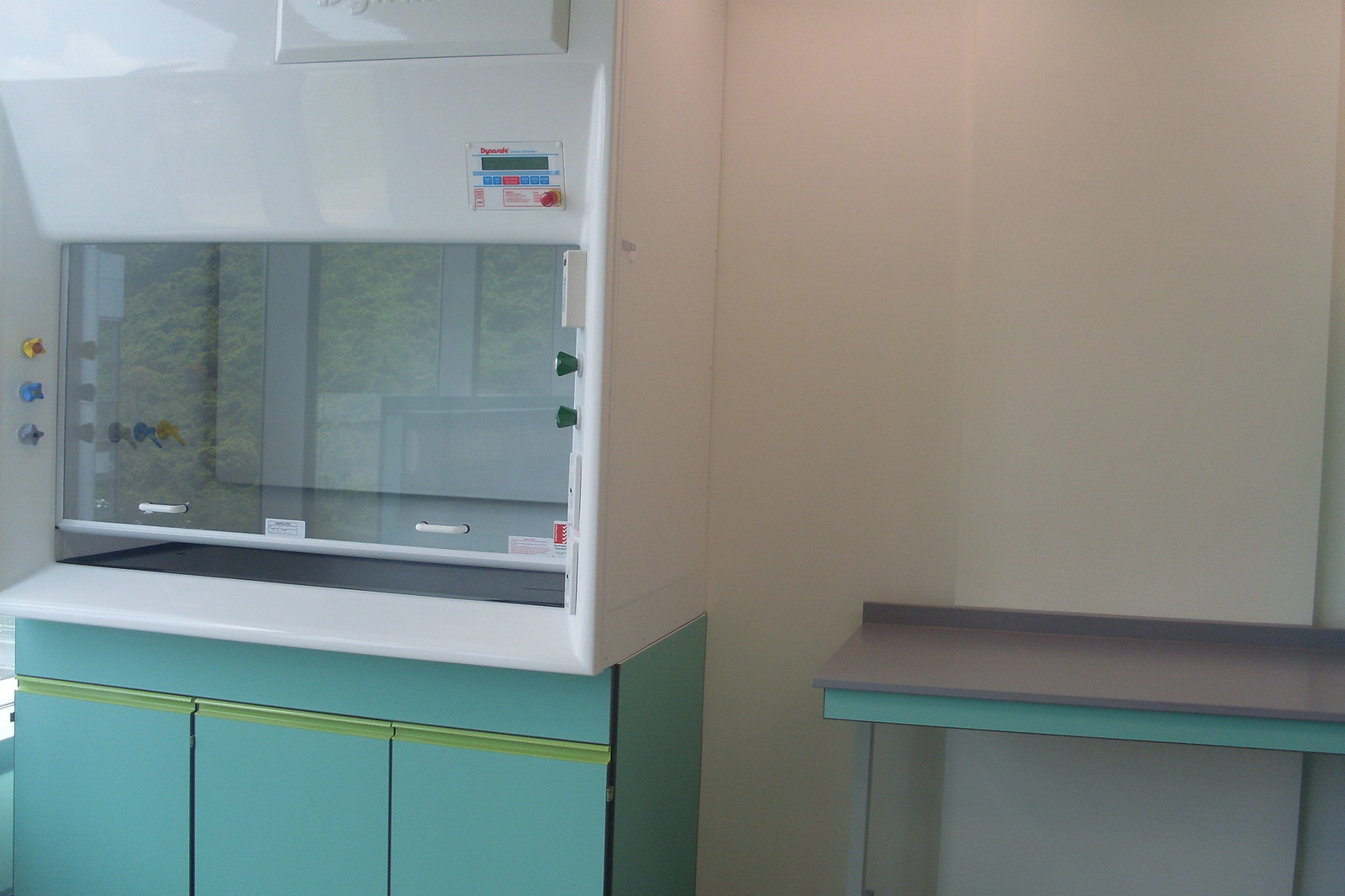This image showcases the interior of what appears to be either a laboratory or a science classroom. Dominating the left side of the photograph is a large, white machine that resembles an incubator or some sort of scientific oven. This machine features a nearly closed glass door, framed by a silver edge at the bottom, and a handle at the top for easy opening. Positioned to the left of the door are three knobs in yellow, blue, and gray, while the right side of the door features two green knobs. Above the glass door is a rectangular digital interface, which includes a screen and a red light indicator, suggestive of temperature control settings.

The machine is placed on top of a turquoise cabinet that has three doors, complete with a noticeable yellow line running horizontally across it. The entire setup—including the white machine and the turquoise cabinet—sits against a beige-colored wall. On the right side of the image, there is a gray tabletop with a turquoise lip underneath, which further suggests its setting within a scientific or educational environment. The combined details—the high-tech equipment, the colorful and organized elements, and the durable furnishings—strongly indicate a functional and instructional space designed for scientific work or learning.